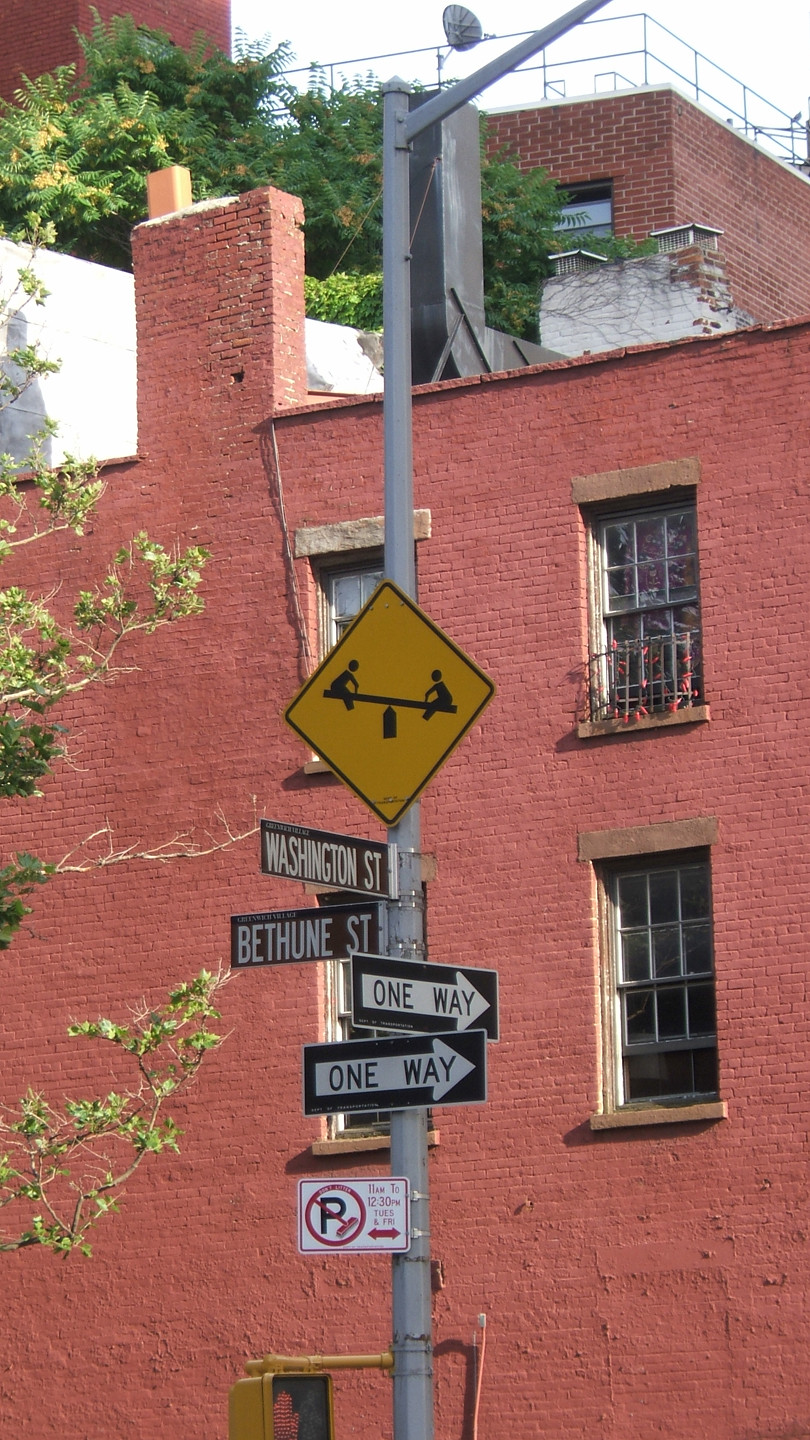This image is a vertically oriented, first-person perspective of a complex array of street signage mounted on a singular cylindrical pole. The central pole is topped with an additional pole that extends diagonally to the right and out of frame, possibly supporting either a traffic light or a street lamp. The signage is organized from bottom to top as follows:

- At the base is a white sign displaying a 'No Parking' symbol: a red circle with a black 'P' in the middle, crossed out by a red line. This sign includes hard-to-read text possibly indicating restricted parking times, which might state "Tuesday and Friday".
  
- Positioned above it is a 'One Way' sign with a right-pointing arrow. This sign features white text on a black background.

- Continuing upward, another 'One Way' sign is visible. This one points straight ahead, its arrow indicating forward direction is evident because the viewer is observing the signs from a slight angle, suggesting they might be standing at a corner.

- Above these, to the left side, is a street sign that reads "Bethune Street" in white text on a green background.

- Above the 'Bethune Street' sign, another street sign points to the left with the name "Washington Street".

- Topping off the array is a yellow cautionary sign depicting a seesaw, potentially indicating a nearby children’s zone or playground.

In the background, there is a red brick building that exhibits signs of wear. Rusted railings are visible around one of the windows, contributing to the building's dilapidated appearance. There are four windows in total, arranged in two rows and two columns. The signage partially obstructs the view of the bottom left and top left windows, while the windows on the right remain unobstructed.